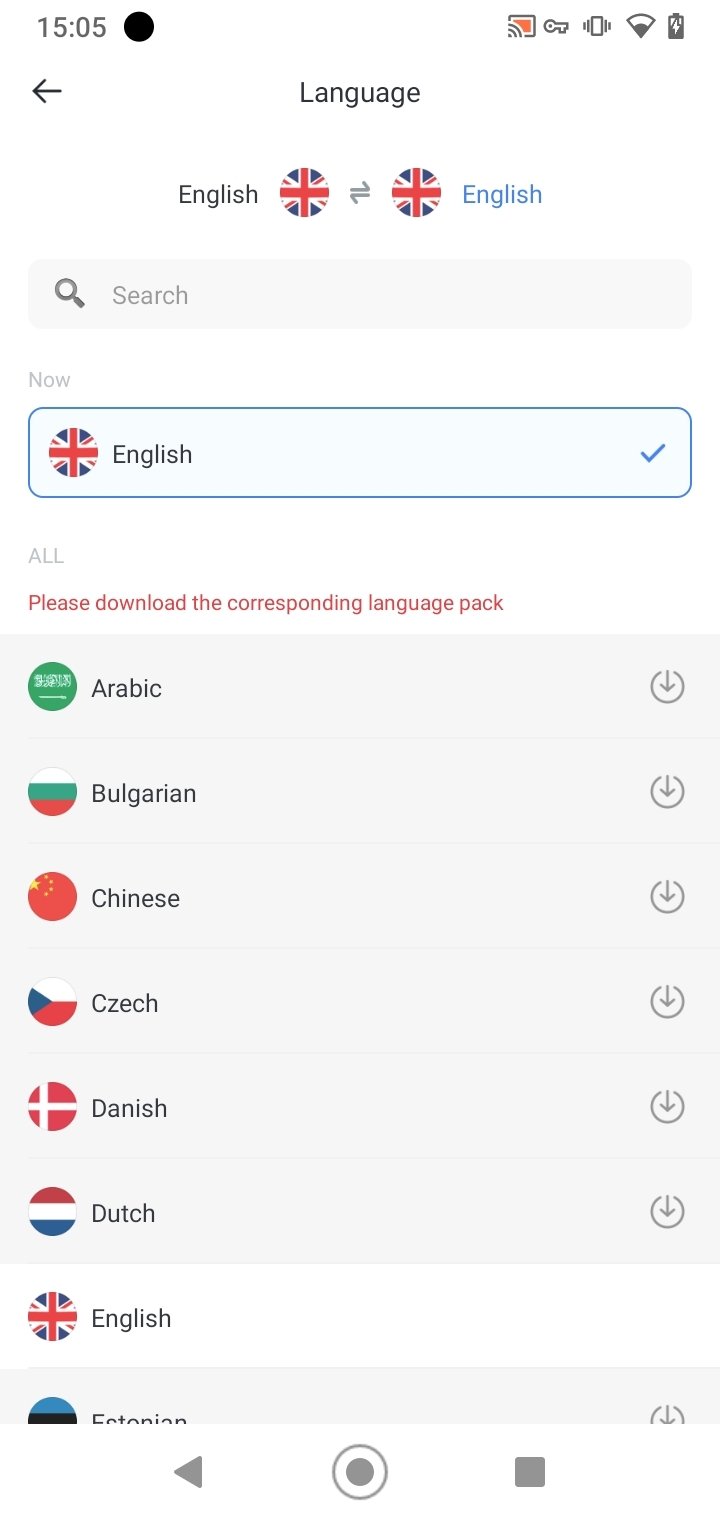This image features a printout detailing various languages selection and options. At the very top, the time "15:05" is displayed within a black oval. To its right, there are five clickable icons. Just below this section, spanning from left to right, an arrow pointing left is seen. Centered at the top of the page is the heading "Language." Beneath this heading, again from left to right and centered on the page, the word "English" is accompanied by the English language logo and two other icons, with the word "English" highlighted in blue.

Following this, there is a search box with a magnifying glass icon on the left side. The word "Search" appears next to it. Adjacent to this is the word "Now," accompanied by the English language icon with the word "English" and a checkmark located at the far right within a blue highlighted box.

Following this section, the word "All" appears, along with a red highlighted sentence that reads, "Please download the corresponding language pack." Below this, various icons represent different languages, listed on the left side as follows: Arabic, Bulgarian, Chinese, Czech, Danish, Dutch, English, and one other language not fully visible. To the far right of these language options, there are downward arrows, presumably serving as clickable references for additional information.